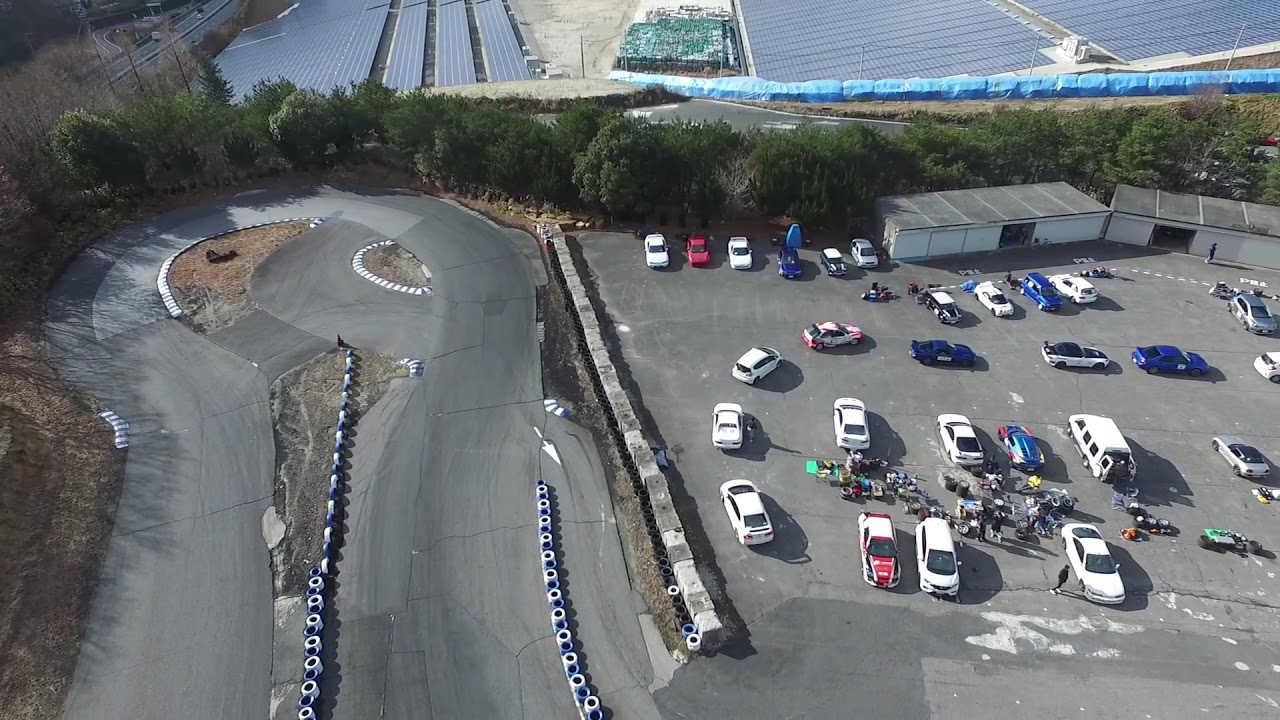The image presents an aerial view of a go-kart racetrack situated on the left side, characterized by a winding course featuring a sharp horseshoe turn. The track is bordered by alternating blue and white tires. Adjacent to the track, on the right, there is a parking lot with approximately 20 cars, predominantly white, with a few blue and red vehicles interspersed. Notably, people appear to be congregating among the parked cars. The entire area, including the track and parking lot, is paved with blacktop. In the background, two large garage-like buildings are visible at the north end, beyond which lies a solar field dotted with solar panels. The northern edge of the image is lined with trees, providing a natural border behind the garages. Despite the absence of active go-karts, tire marks are prominently visible, particularly around the horseshoe turn, indicating previous activity on the track.